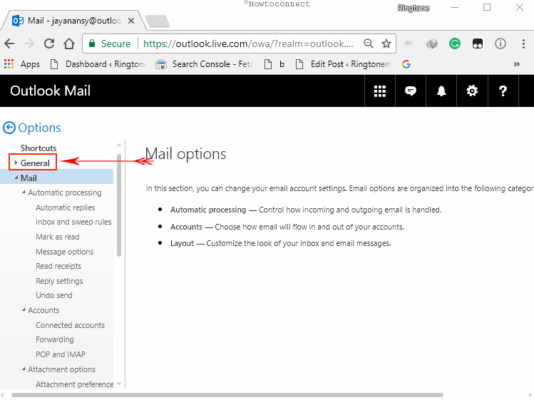This image depicts a detailed view of a web page interface, specifically within the Outlook Mail service. At the top of the page, the title reads "Mail Jayan's Outlook". Below the title bar, there's a browser tab with navigation arrows pointing left and right, as well as refresh and home icons. 

Moving down, there's an address bar displaying the website address. Below the address bar, a black banner is present, prominently displaying "Outlook Mail" along with a set of icons aligned to the right side.

Further down the page, a sidebar menu is visible on the left side. Within this sidebar, the "Options" link is highlighted in blue. Underneath this, there are several menu items categorized as "Shortcuts" and "General", with the "General" category highlighted with a red border and a red arrow pointing to it.

Adjacent to this, a blue banner is visible, marked with the label "Mail". Beneath the blue banner, there is another section listing various mail management options including "Automatic Processing", "Automatic Replies", "Inbox and Sweep Rules", "Mark as Read", "Message Output Options", "Read Receipts", "Reply Settings", "Undo Send", "Accounts", "Connected Accounts", "Forwarding", "POP and IMAP", "Attachment Options", and "Attachment Preferences".

In the central part of the page, the header "Mail Options" is displayed. Below this header, a message explains that users can change their email account settings and that email options are organized into categories such as Automatic Processing, Accounts, and Layout.